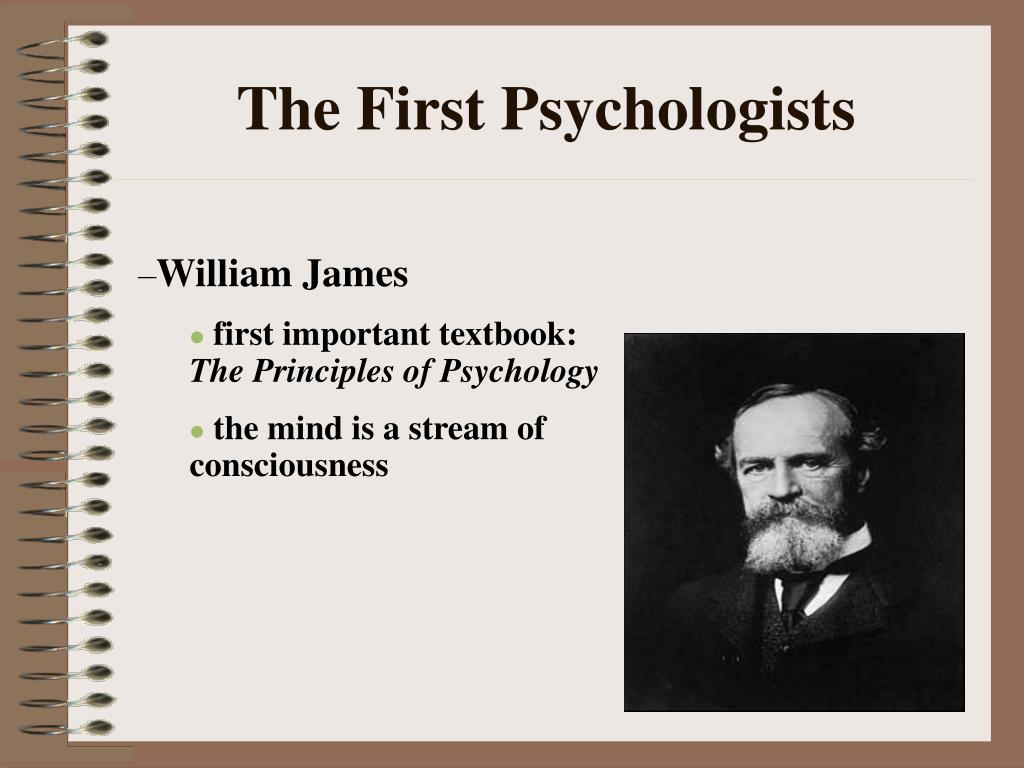The image depicts a page from a loose-leaf binder with a brown background and visible metal rings on the left-hand side. The page features the heading "The First Psychologists" in brown print, followed by a thin line. Underneath, in black capital letters, it reads "William James" with a dot below it. The next line states "First Important Textbook: The Principles of Psychology" in italicized text, followed by another dot. Below that, it says, "The Mind is a Stream of Consciousness." On the bottom right corner of the page, there is a black-and-white photograph of William James, an older gentleman with dark hair and a white beard, dressed in a three-piece suit and tie. The overall layout appears to be part of a slideshow slide with a notebook theme and a brown background.